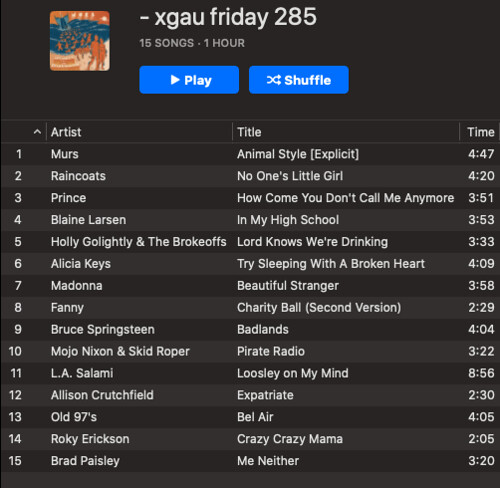This is a detailed screenshot of a music playlist. The background of the image is black. In the top left corner, there is a square photo of an album cover. To the right of the album cover, the text "Dash X GAU Friday 285" appears in large white letters. Below this, in small gray letters, it reads "15 songs, 1 hour."

Centered on the page are two buttons: a "Play" button and a "Shuffle" button. Both buttons are blue with white text.

Directly below these buttons, the column headers "Artist," "Title," and "Time" are listed from left to right. Each header is followed by a vertical list of corresponding information.

Under the "Artist" column, the first entry is "MERS" with the corresponding title "Animal Style (Explicit)" and a duration of "4:47" under the "Time" column. 

The second entry lists "Raincoats" as the artist, with the title "No One's Little Girl" and a duration of "4:20."

The third entry lists "Prince" as the artist with the title "How Come You Don't Call Me Anymore" and the duration "3:51."

This pattern continues down, listing a total of 15 songs.